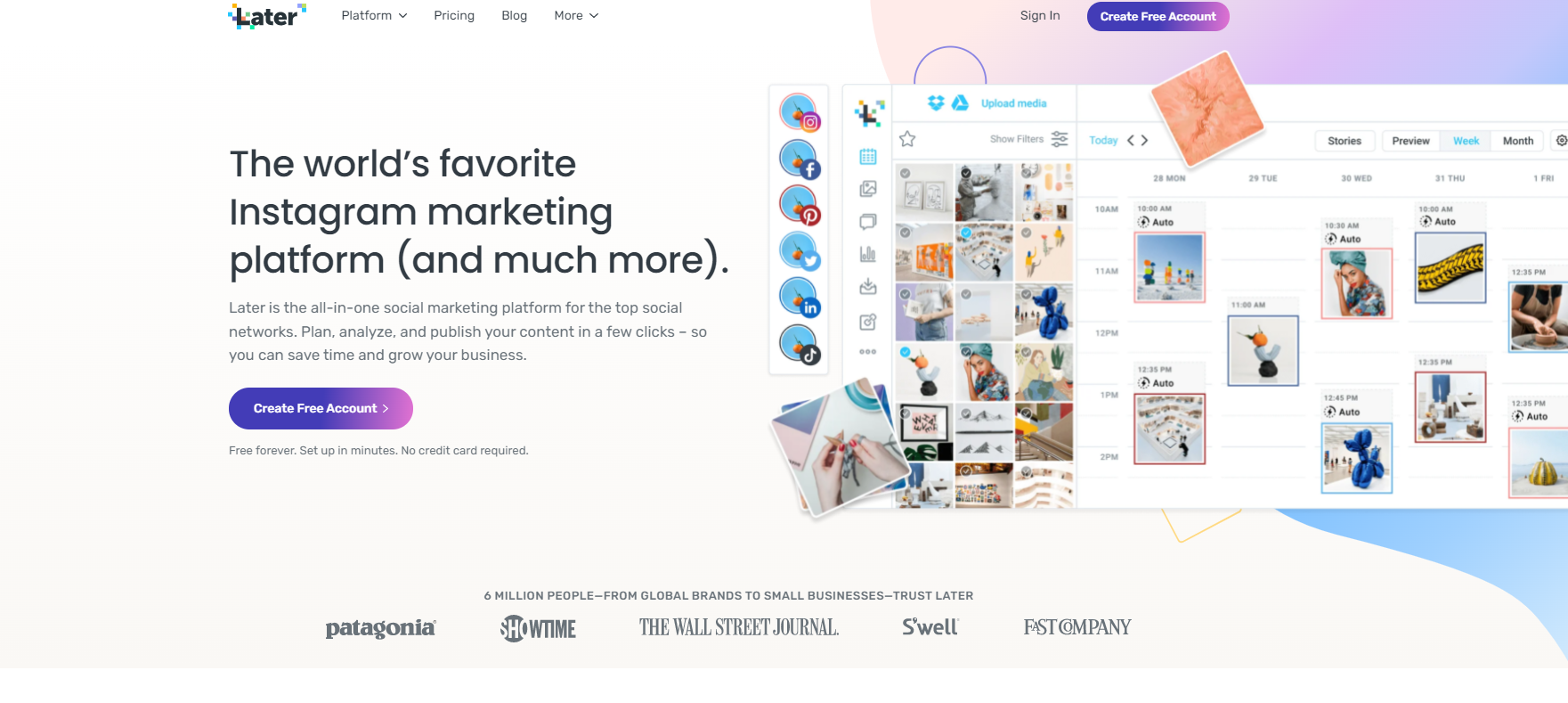The image appears to be a screenshot of a website called "Later," as indicated by the text in the top left corner. The website features a navigation bar with dropdown options for "Platform," "Pricing," "Blog," and "More." A prominent headline on the left-hand side declares "The World's Favorite Instagram Marketing Platform (and much more)," positioning Later as an all-in-one social marketing solution for major social networks. The text explains that Later enables users to plan, analyze, and publish content with just a few clicks, helping them save time and grow their business.

Underneath this description is a noticeable, clickable button that reads "Create Free Account," accompanied by reassurances such as "Free forever," "Set up in minutes," and "No credit card required." 

On the right side of the image, there are visual representations of what the platform's dashboard looks like, showing links for Instagram, Facebook, Pinterest, Twitter, and Indeed, along with another icon that is not easily identifiable. The site also offers options to "Sign In" or "Create Free Account" at the top.

Displayed in the dashboard preview are examples of how videos or images would appear on the platform. Additionally, a calendar feature on the right allows users to schedule content for future publication dates. 

The bottom section of the image highlights a trust statement: "Six million people, from global brands to small businesses, trust Later." Beneath this statement are affiliate links featuring logos of well-known organizations like Patagonia, Showtime, The Wall Street Journal, Swell, and Fast Company.